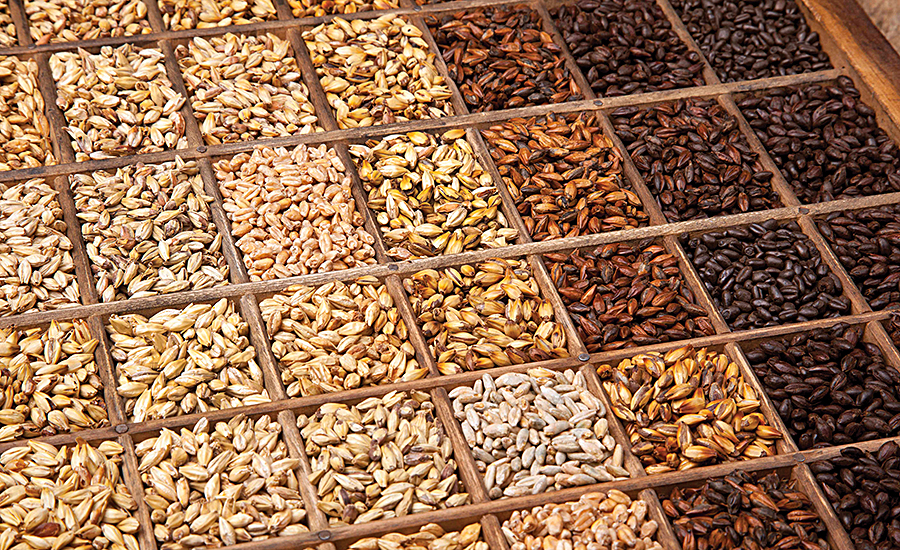This landscape-oriented image features a close-up of various nuts, seeds, and coffee beans meticulously organized in a grid of wooden compartments. The compartments are created by thin horizontal and vertical wooden dividers, forming numerous small square sections. On the far left, the compartments contain lighter-colored nuts and seeds, potentially sesame seeds or unroasted pistachios. As your eyes move towards the center, the contents transition into golden and brown hues, indicating varying degrees of roasting or different types of nuts. On the far right, the compartments display dark brown, almost black items, which are clearly roasted coffee beans. The arrangement visually progresses from light to dark, emphasizing the different stages of roasting or types of seeds and nuts. There are no people or text in the image, drawing full attention to the carefully sectioned and color-graded assortment of beans, nuts, and seeds.